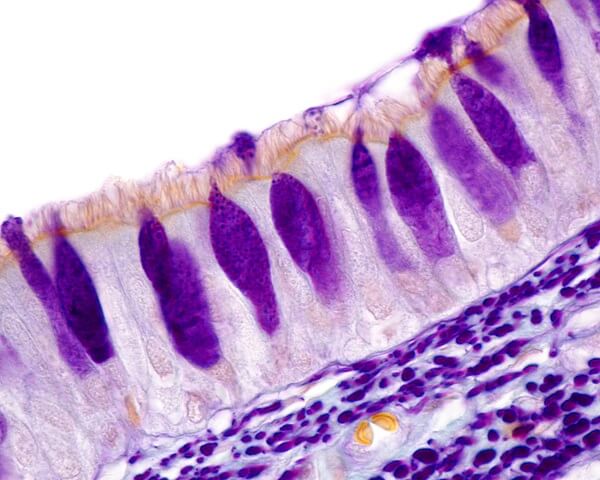The image resembles a scientific illustration with a multitude of purple hues, ranging from dark purple, light purple, lavender, to violet. The top left portion of the image is a blank, untouched white space. Below this, there's a light brown string or line that starts about halfway down the right side and curves slightly upwards towards the top quarter. This light brown line is decorated with purple, fish-shaped objects, which could also be interpreted as teardrops, closely spaced along its length.

Adjacent to this line is a region filled with elongated, oval or ovoid-shaped dark purple blobs. These blobs appear vertical or diagonal, running from near the top to the bottom of the lighter purple section, numbering around 12 or 13 in total.

Below these vertically aligned structures, there's an area densely packed with smaller, darker purple globules or dots, interspersed with some very small round orange and yellow spots. These could be interpreted as nuclei within cells, contributing to the impression that the image contains cellular structures and tissue types. The entire painting is bordered by a purplish-pink frame, intensifying the vivid and somewhat abstract representation evocative of biological microscale elements.